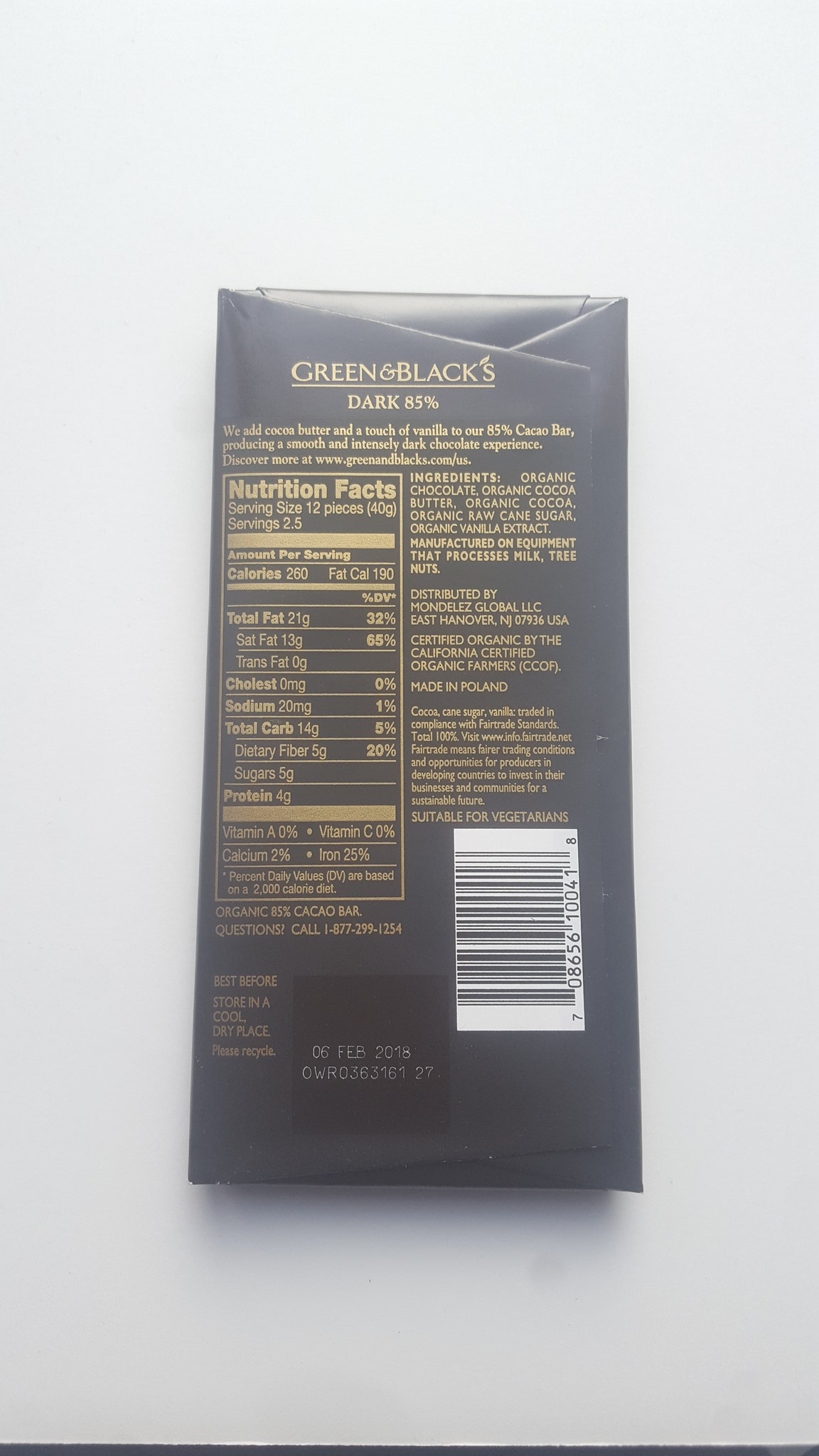The image showcases the detailed back view of a Green & Black's Dark 85% Chocolate bar package. The wrapper, made of black paper, is meticulously folded and glued, creating a sleek and elegant design. Prominently displayed is a white UPC barcode with black lines and corresponding numbers beneath it.

The text on the package prominently features the brand's logo and product name, reading "Green & Black's Dark 85%." Below, a brief description informs consumers that the bar includes added cocoa butter and a touch of vanilla to produce a smooth and intensely dark chocolate experience, inviting them to discover more at www.greenandblacks.com.us.

A comprehensive Nutrition Facts panel reveals key dietary information: a serving size is 12 pieces (40 grams), with approximately 2.5 servings per package. Each serving contains 260 calories, of which 190 are from fat. The panel further breaks down nutritional content, detailing the amounts of total fat, cholesterol, sodium, total carbohydrates, protein, and various vitamins and minerals.

The list of ingredients emphasizes the product's organic nature, including organic chocolate, organic cocoa butter, organic cocoa, organic raw cane sugar, and organic vanilla extract. Additional information notes that the chocolate is manufactured on equipment that processes milk and tree nuts, catering to those with allergies.

Lastly, the expiration date is clearly printed as 06 February 2018, ensuring consumers are informed of the product's freshness.